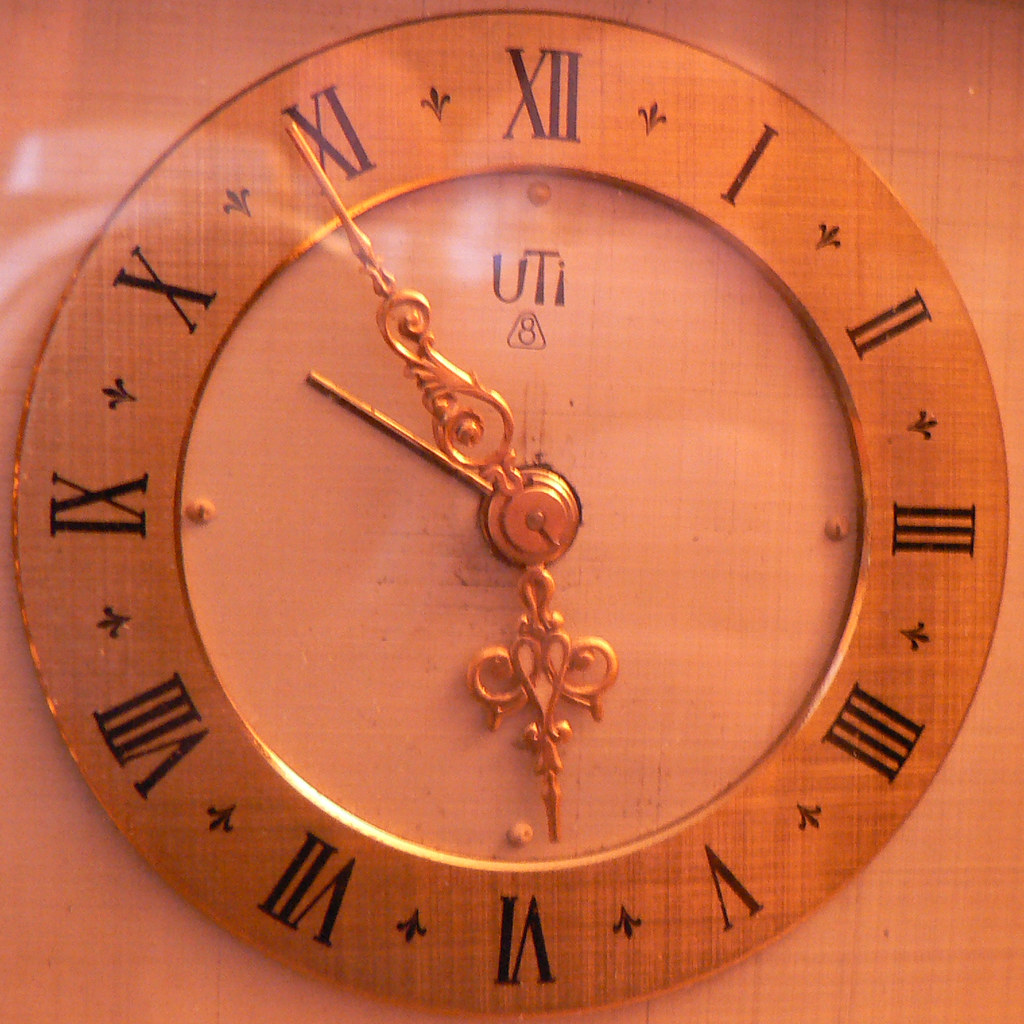This photograph captures a detailed and aesthetically pleasing analog clock hanging on a wall with a peach-colored background, possibly cloth. The clock is characterized by its round shape and a thick frame of orangish wood, where Roman numerals from I to XII are displayed in bold black. Each numeral is separated by a small design, likely a fleur-de-lis symbol. The interior of the clock features a clear, possibly plastic or acrylic face with four visible screws at the 12, 3, 6, and 9 o'clock positions. The clock hands are ornate gold pieces, with the hour and minute hands featuring intricate scrollwork that forms a heart shape before tapering to a point. The second hand is a simple, slender gold stick with a blunt end. The tan-goldish hue of the clock's face adds to its vintage aesthetic, marked by the letters "UTi" at the top and a figure-eight inside a triangle below them. The time on the clock reads approximately six minutes to six. The overall composition of the image highlights the clock's intricate craftsmanship and elegant design.